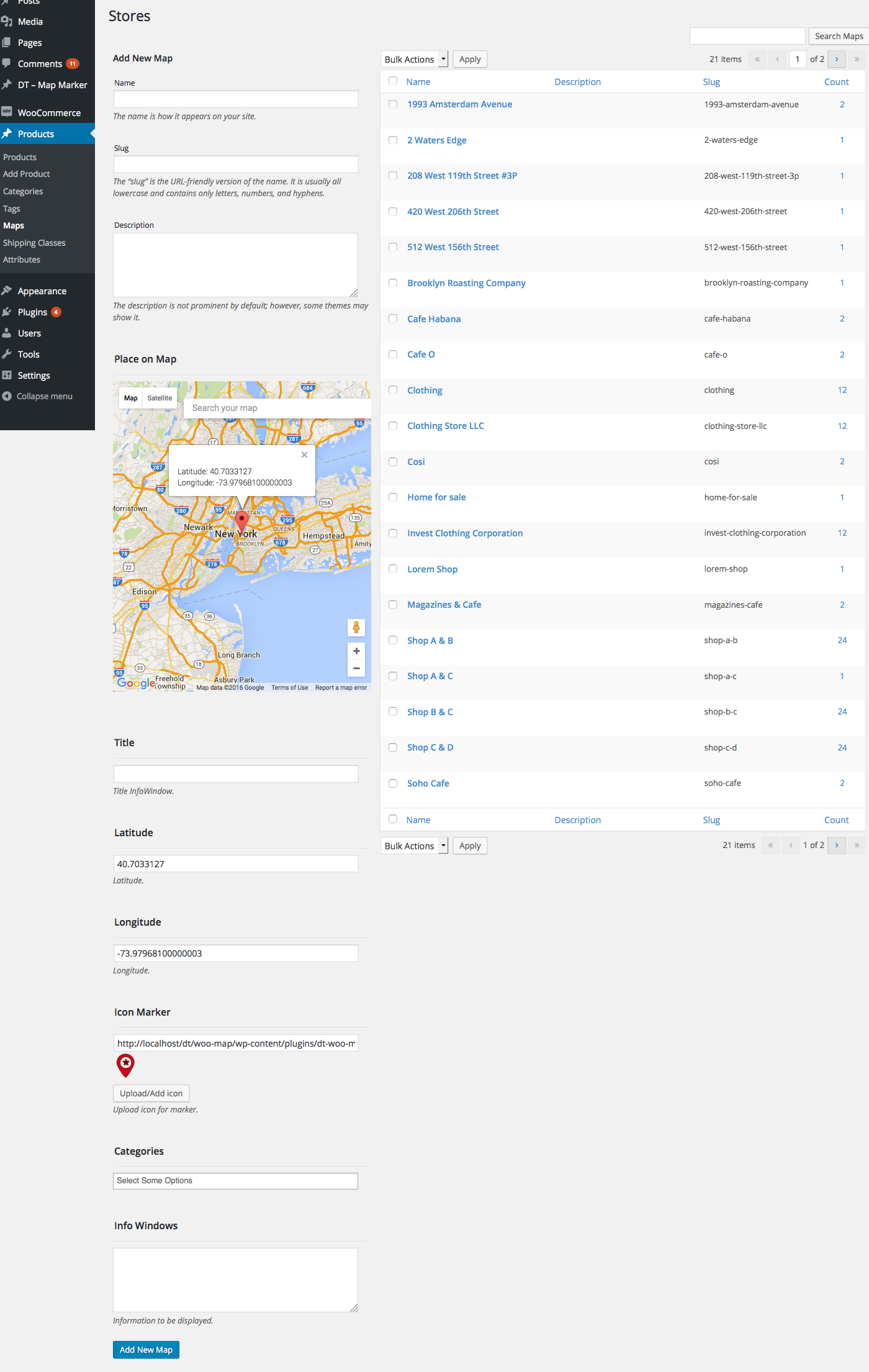The image appears to depict a detailed user interface of a website, likely related to geo-locating or mapping functionalities. In the upper left-hand corner, there is a black, vertical box occupying approximately 10% of the screen space. This box contains an estimated 15 to 20 clickable options. To the right of this section, there is a label that likely reads "Store," followed by a search box where users can presumably input a store name. Below the search box is the text "Places on Map," with a corresponding map image that appears to depict New York City, potentially focusing on Manhattan. Beneath this map section, there are input fields for a title, as well as latitude and longitude coordinates. On the right-hand side of the interface, there are multiple pull-down menus and various selectable options, the specifics of which are unclear due to the small font size.